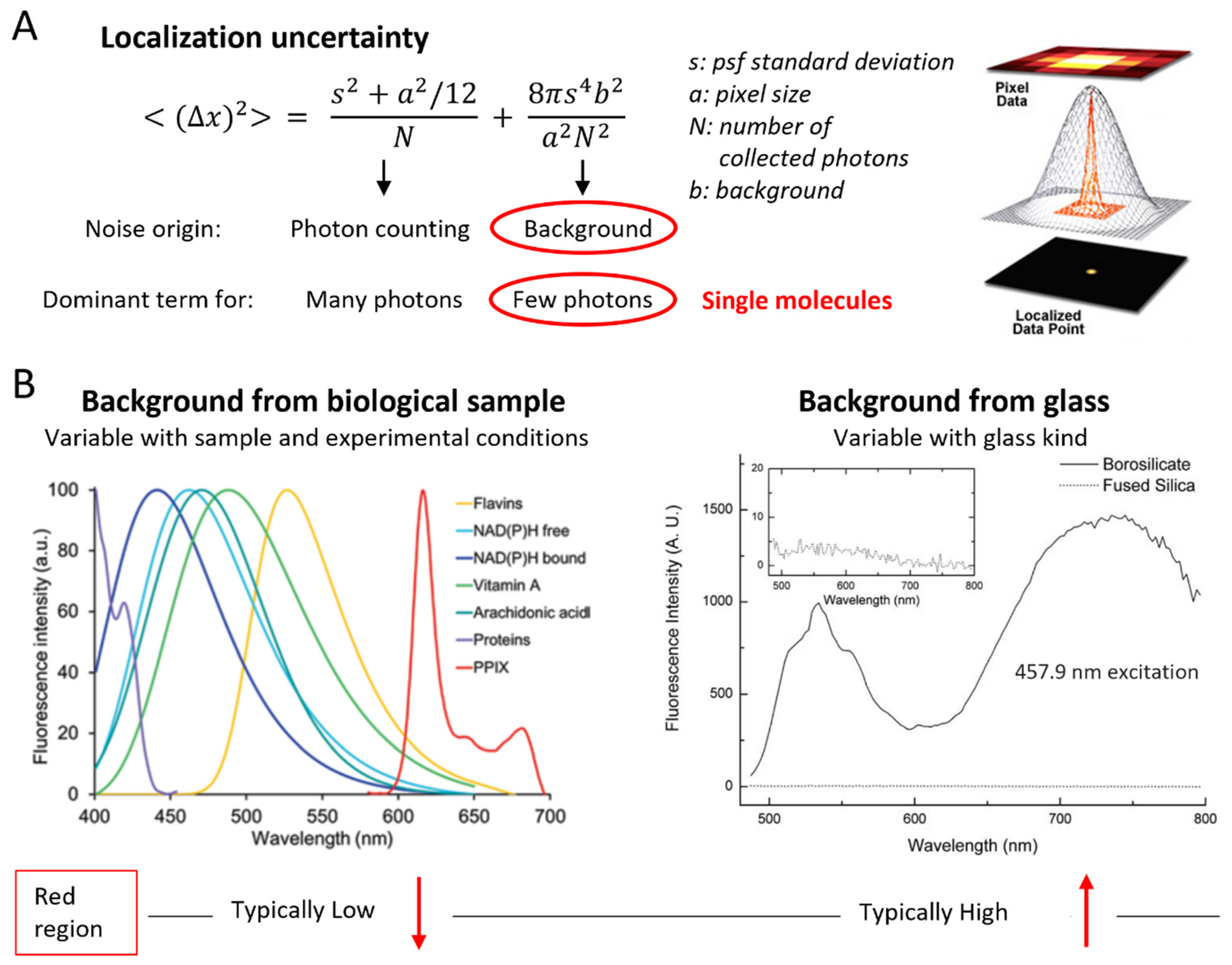The image is a detailed scientific diagram focused on photons and molecules, potentially from a biology textbook. In the upper left corner labeled 'A,' it details "Localization Uncertainty," accompanied by a complex mathematical equation. Beneath this, the terms "Noise Origin," "Photon Counting," and "Background" are mentioned, with "Background" circled in red. Further down, it references "Dominant Term for Many Photons" and "Few Photons," with "Few Photons" also circled in red. To the right, it lists "S: PSF Standard Deviation," "A: Pixel Size," "N: Number of Collected Photons," and "B: Background," followed by "Single Molecules" in red lettering. Adjacent is a diagram featuring "Pixel Data" and "Localized Data Point," showing a cone-like structure below these labels.

The lower section is labeled 'B' and presents two charts. The first chart, titled "Background from Biological Sample, Variable with Sample and Experimental Conditions," has a vertical scale from 0 to 100 indicating fluorescence intensity (AU) and a horizontal scale from 400 to 700 nanometers for wavelength. The chart includes a legend detailing various substances such as flavins, NADPH-free, NADPH-bound, vitamin A, arachidonic acid, proteins, and PPIX. The second chart, titled "Background from Glass, Variable with Glass Kind," contrasts borosilicate and fused silica. It has a vertical scale from 0 to 1500 fluorescence intensity (AU) and a horizontal range from 500 to 800 nanometers. An additional inset graph has a vertical scale from 0 to 20 and a wavelength range from 500 to 800 nanometers, highlighting a line at 457.9 nanometers excitation. At the bottom, there is a red-boxed label "Red Region," indicating "Typically Low" with a downward red arrow and "Typically High" with an upward red arrow.